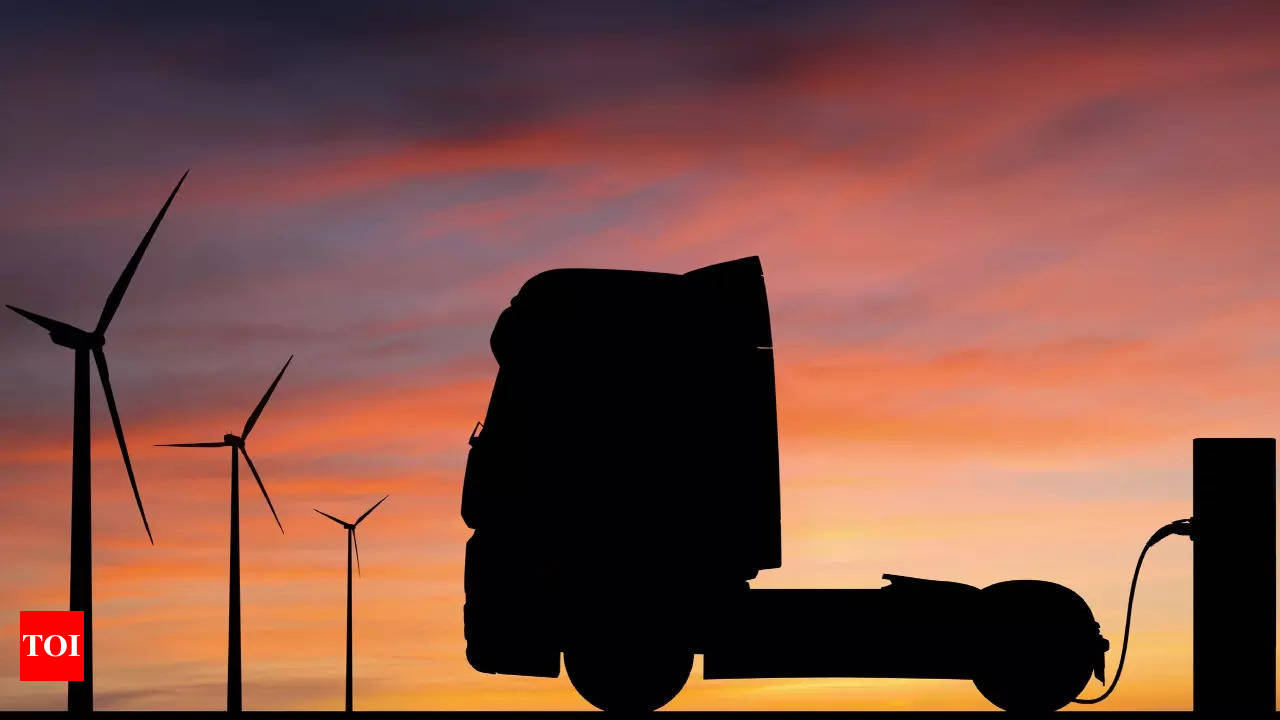In this evocative image, three towering windmills with tri-pronged blades stand silhouetted in the left corner against a beautiful, multicolored sky that transitions from blue and pink at the top to shades of orange, yellow, and a pale gray near the horizon. In the foreground is the dark silhouette of what appears to be an electric semi-truck, typically used for towing large trailers, connected to an electric charging station, emphasizing the theme of renewable energy. A hose links the truck's flatbed to the charging station, underscoring the transition to sustainable transportation. The serene, rural backdrop lacks other geographical features, keeping focus on the green energy elements. At the bottom left corner, a small red square contains the white letters "T-O-I," likely indicating the image’s source from a media outlet.